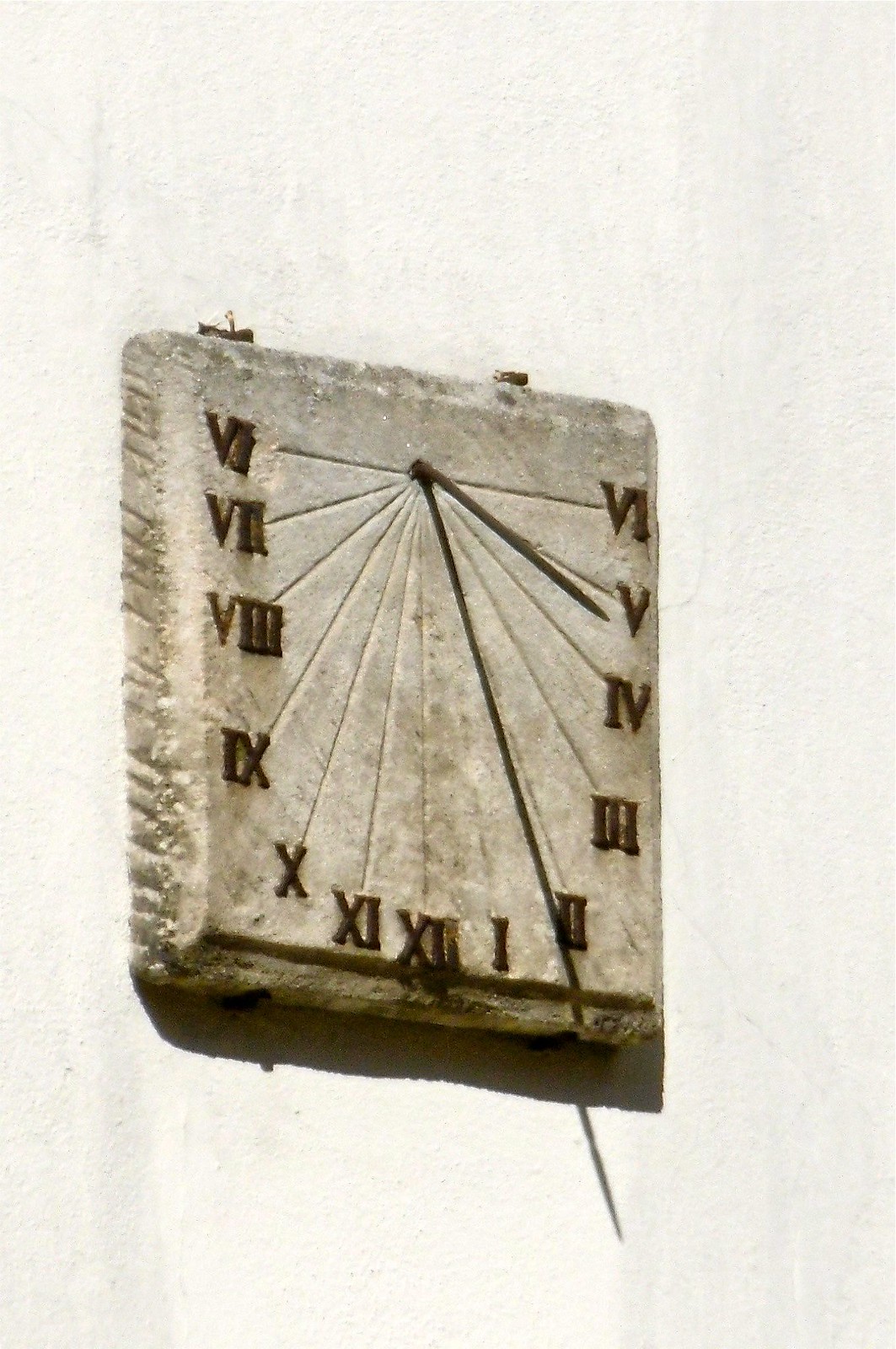This is a monochromatic image depicting a concrete square mounted on a wall. Intriguingly reminiscent of a Roman numeral clock, it features an array of engraved numerals arranged in a U-shaped pattern. Starting at the top right corner with the numeral VI (6), the sequence continues with V (5), IV (4), III (3), II (2), I (1), XII (12) at the bottom center, and then curves back upward with XI (11), X (10), IX (9), VIII (8), VII (7), and concluding back at the starting point with VI (6) at the top left. 

At the top center of the square, two sticks—one shorter and one longer—protrude, resembling clock hands. Radiating from this central point, engraved lines fan out towards each numeral, enhancing the clock-like appearance. The image is bathed in bright light, casting a harsh shadow beneath the structure, which amplifies the textures and details of the concrete. The color palette is primarily grayscale with a hint of red, suggesting a desaturated aesthetic that almost mimics a black-and-white photograph with the exclusion of blue hues.